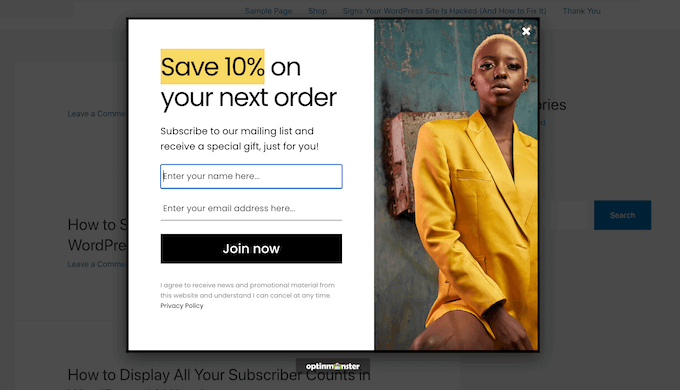The image depicts a pop-up advertisement on a clothing sales website. The pop-up prominently features an offer to "Save 10%" on your next order, highlighted in yellow. It encourages visitors to subscribe to the mailing list with the promise of a special gift. The form within the pop-up includes a rectangular text box labeled "Enter your name here," followed by a line above which it reads "Enter your email address here." Below this is a black rectangular "Join Now" button with white text, and beneath it is a statement: "I agree to receive news and promotional material from this website and understand I can cancel at any time," accompanied by the words "Privacy Policy."

To the right side of the pop-up, there is an image of an African-American woman with very short hair, wearing a mustard yellow outfit and looking directly at the camera with a neutral expression. The background behind her is a blend of colors without any distinct image, giving it a modern, abstract appearance. An "X" in the upper right corner allows users to close the pop-up.

The pop-up partially obscures the underlying webpage, making it challenging to see its contents. However, a small portion at the bottom of the main page is visible and reads, "How to display all your subscriber counts." Other details of the underlying page remain unclear due to the dominance of the pop-up.